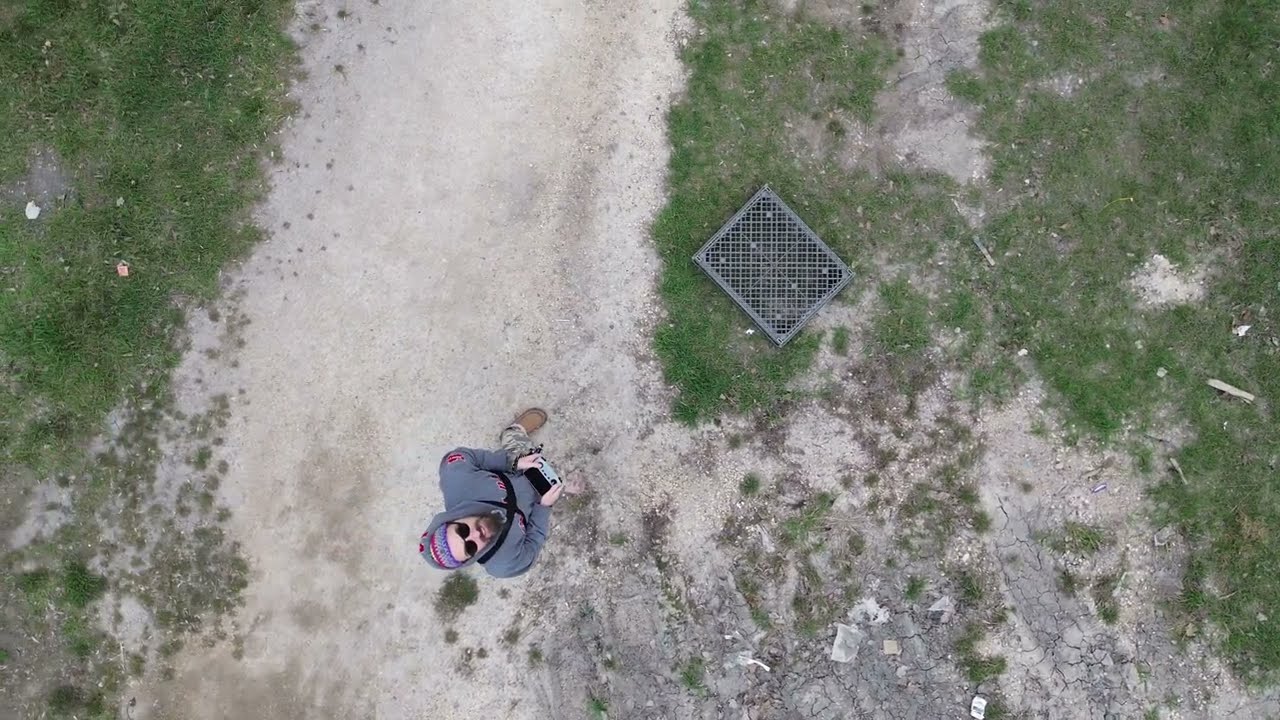In this overhead shot, a white man with facial hair, possibly a beard or goatee, stands on a dirt pathway surrounded by sparse green vegetation, grass, and rocks. He is looking up directly at the camera, which may be a drone he is operating. The man is wearing a gray hoodie over a beanie and sunglasses, along with camouflage-colored pants and tan boots. Visible strapped across his chest is a crisscross formation of straps, likely for his drone controller. He appears to be holding a remote control, suggesting he is indeed a drone operator. In the background, a gray object, possibly a milk crate, serves as a makeshift landing pad for the drone. The environment around him looks quite desolate.